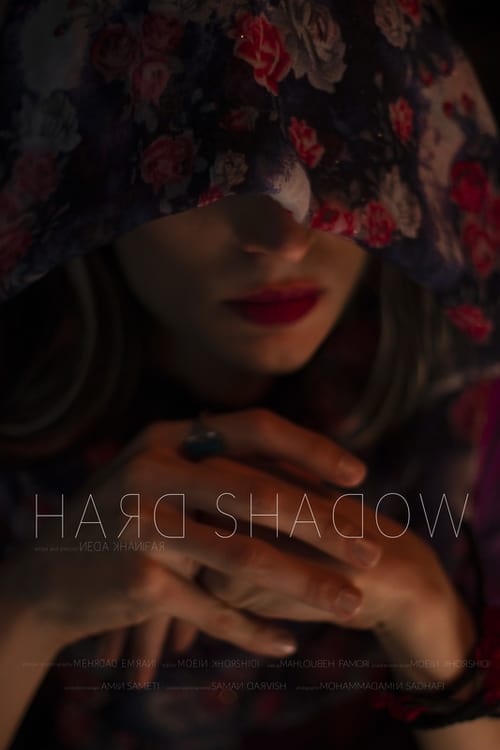The image is a dark, shadowy movie poster titled "Hard Shadow," with the R and D in both words printed backwards, suggesting a mysterious, possibly a murder-mystery theme. The photograph is rectangular, with the central figure being a woman who appears pensive. She is sitting and facing the camera, her attentive pose accentuated by hands clasped in front of her, one over the other, adorned with a ring. She wears a pinkish-red lipstick and a fabric, possibly a scarf or bandana, covers the upper part of her head, including her eyes, but her nose and mouth remain visible. The scarf has a floral decoration, adding a touch of delicacy to the somber shades of pink, silver, white, black, olive, gray, and red in the image. Soft, candle-like lighting illuminates her face and hands, creating a captivating contrast against the eerie darkness of the background. Additional text, difficult to decipher due to the shadows, is also present on the poster, contributing to the overall enigmatic feel.